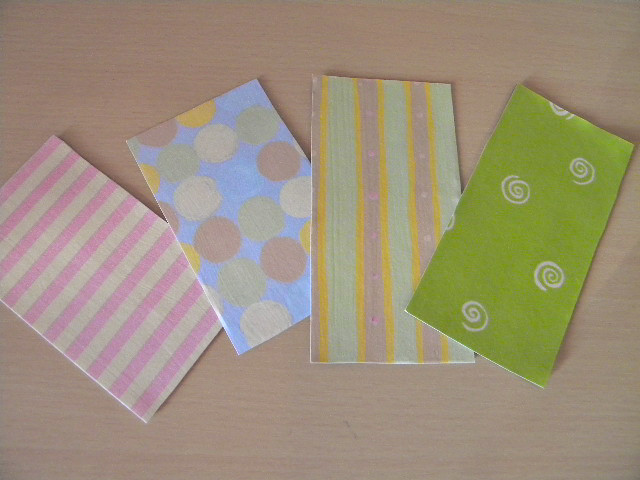The image is a detailed color photograph featuring four rectangular swatches, fanned out in a barely overlapping manner on a pale gray textured background. These swatches appear to be samples of decorative wallpaper or thick decorative paper with a fabric-like appearance. Each piece is meticulously cut from larger rolls, designed to enhance interior spaces.

From left to right, the swatches display unique patterns and colors:

1. The first swatch features pink and off-white horizontal stripes with wavy edges that add texture and visual interest.
2. The second showcases a light blue background adorned with large polka dots. The dots come in various brush stroke-like hues, including white, light green, tan, yellow, and blue.
3. The third is characterized by vertical stripes in a subtle mauve or purple shade with small white dots. This central stripe is bordered by thin yellow stripes and, further out, by light cucumber green stripes.
4. The final swatch displays a bright grassy green background interspersed with white spirals, of which four full spirals are prominently visible, along with partial spirals peeking from the edges.

The arrangement and diverse patterns in these colorful swatches project a vibrant and eclectic aesthetic, suitable for a range of decorative applications.